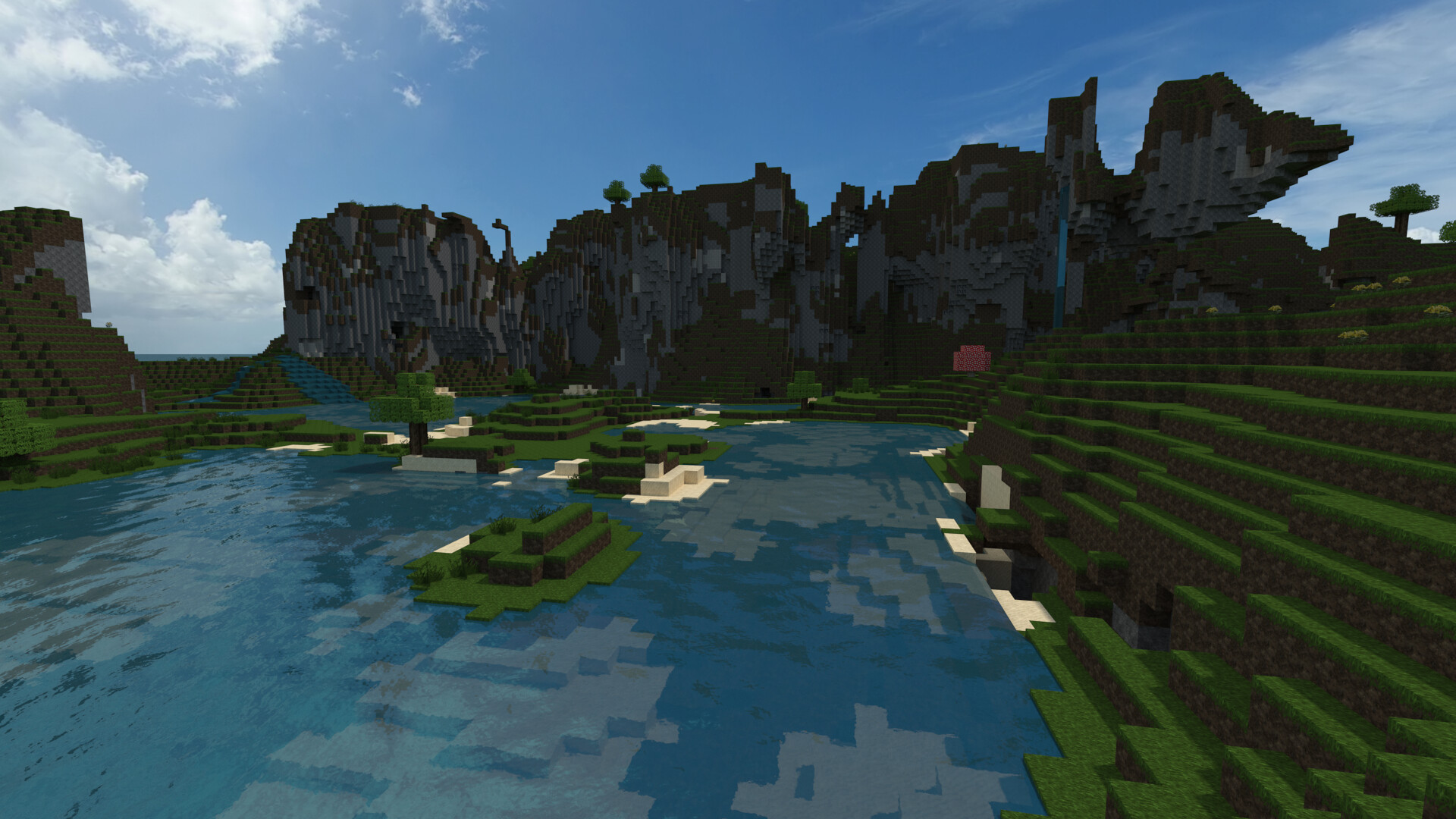The screencap from the game Minecraft showcases a vibrant, blocky landscape with a variety of natural elements and terrain. In the foreground, a dark blue pond mirrors the white clouds from the cyan sky above. The water appears shallow, revealing submerged, light gray blocks that form a textured bed. Scattered across the water are dark green floating islands, some edged with dark brown cliffs and topped with green grass, which include highlights of light tan sand. On the left side of the image, a larger island stands out with its lush greenery, dark brown soil, and a blocky dark green tree. This island features a series of steps that ascend towards the sky. 

The central part of the image is dominated by a towering mountain composed of various shades of dark and light gray blocks, accented by patches of dark brown and green. The mountain's rugged terrain continues into the distance, blending into other peaks that mix gray rock and brown dirt, with occasional trees crowning their summits. 

To the right, a small square section seemingly filled with red and pink blocks suggests a building-like structure, providing a vivid contrast to the surrounding natural landscape. Further right, another green shelf topped with dark brown dirt rises in tiers, populated by additional trees. This intricate scene, captured in a pixelated, digital art style reminiscent of 8-bit or 16-bit visuals, emphasizes the layered, modular beauty of the Minecraft world.